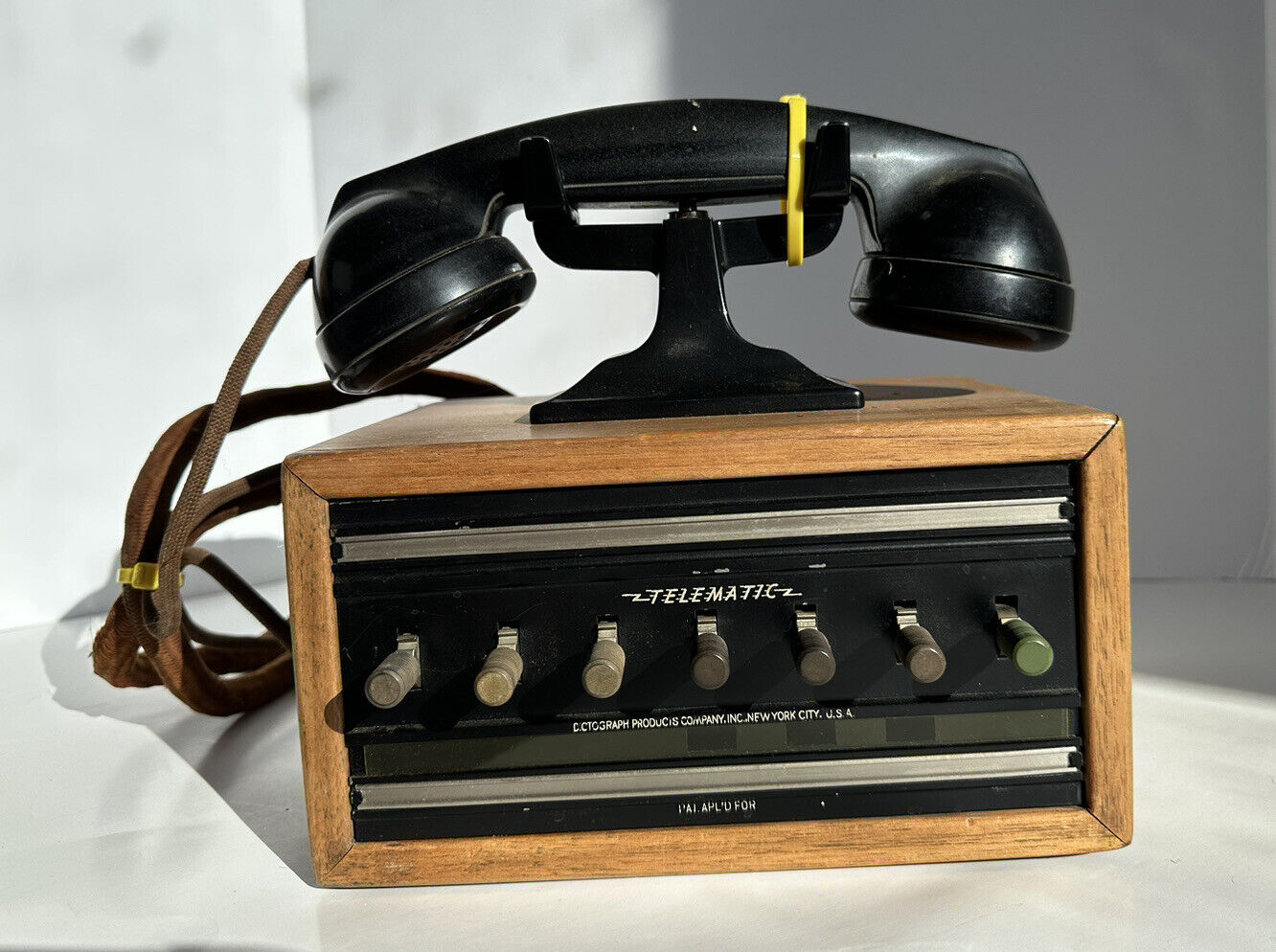This is a horizontal image of a vintage telephone, prominently featuring a black receiver resting on its cradle, which is mounted atop a wooden box. The black telephone cord, appearing to be leather and secured with a yellow zip tie, adds to its antique charm. This wooden box functions as a mechanical device with seven turnable knobs protruding from the front, arranged from left to right. Above the knobs, the word "Telematic" is inscribed, with "New York City" written underneath. The entire setup, including the black holder and knobs, is positioned on a white surface, against a backdrop of white walls, emphasizing its historic and retro characteristics.